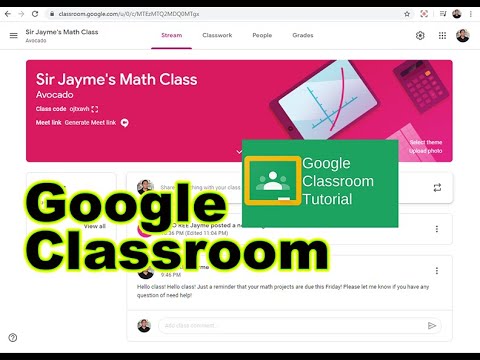The image displays a screenshot of a Google Classroom interface for Sir Jamie's math class. The layout features typical classroom supplies such as a calculator, paper, and specifically graph paper, which are integral for math projects. Prominently, there is a large red rectangle inside the image, beneath which is labeled "Avocado Class Code" and "Meet Link," indicating a link for online meetings. Additionally, there is a box marked "Google Classroom Tutorial" with the text "Google Classroom" in bold black letters, outlined in yellow, making it highly noticeable. The URL "classroom.google.com" is visible in the search bar at the top of the screen. At the bottom of the image, a message is discernible: "Hello class, hello class. Just a reminder that your math projects are due this Friday. Please let me know if you have any questions or need help." This message is designed to prompt student responses in the space provided.